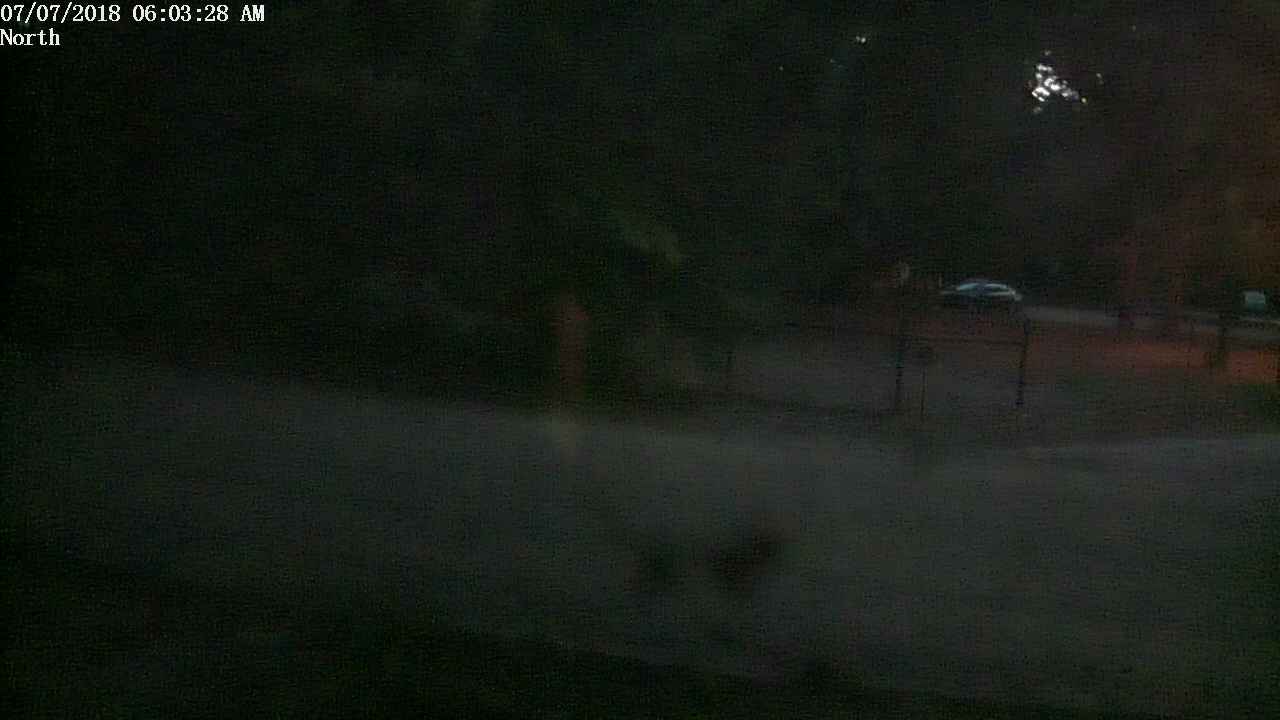The image appears to be a blurry, dark photo taken from security footage, timestamped in the top left corner with "07/07/2018 6:03:28 a.m." and marked "north." The scene is an outdoor environment, likely at dawn, as suggested by the medium dark blue sky and faint sunlight. The main focus is a street flanked by trees, a fenced area, and a field, possibly grass or a mowed cornfield. A dark-colored car, potentially in a parking lot, is visible in the background. In the foreground, a blurry figure, likely a dog based on the visible tail and body shape, is walking down the street. Further back, a house might be partially obscured by the trees, and faint red light appears to emanate from the right-hand side.